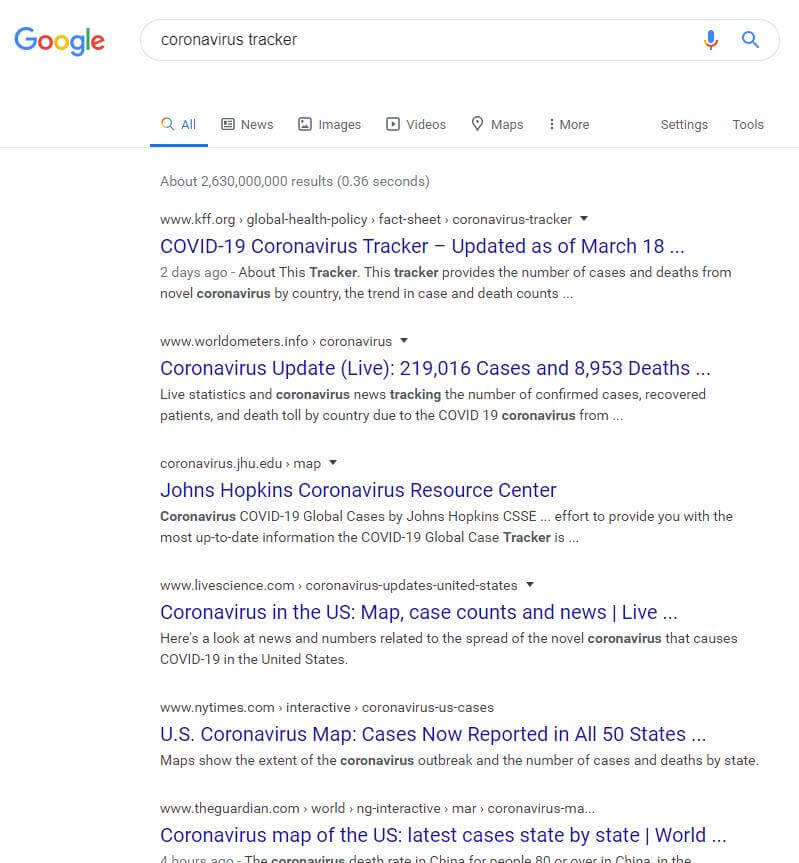The Google search results page prominently displays the Google logo in the upper left corner with its distinctively colorful letters. In the central search bar, the user has typed "coronavirus tracker." Adjacent to the search box, there is a microphone icon and a magnifying glass graphic symbolizing voice search and the search functionality respectively. Immediately below the search bar, a menu provides various options including "All," "News," "Images," "Videos," "Maps," "More," "Settings," and "Tools." 

Displayed prominently below this menu are the search results, indicating approximately 2.63 billion results found in 0.36 seconds. The top result is titled "COVID-19 Coronavirus Tracker - Updated as of March 18," followed by an ellipsis, and it is hosted on the website www.kff.org. The listing contains a breadcrumb trail indicating navigation options: Global Health Policy > Fact Sheet > Coronavirus Tracker.

Subsequent entries include:

1. "Coronavirus update live" from John Hopkins.
2. "John Hopkins Coronavirus Resource Center."
3. "Coronavirus in the U.S.: Map, Case Counts, and News."
4. "U.S. Coronavirus Map: Cases Now Reported in All 50 States."
5. "Coronavirus Map of the U.S.: Latest Case Count by State and Worldwide."